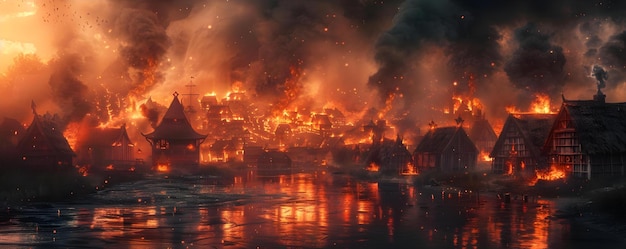This striking nighttime image captures a chaotic scene where a large fire engulfs a town, casting an ominous glow across the landscape. The horizontally aligned rectangular photograph showcases a broad swath of flames stretching from the left to the right, consuming rows of wooden houses. In the upper half of the image, thick, dark plumes of smoke ascend into the night sky, with a particularly bright area of flames illuminating the upper left corner. The brightness diminishes towards the right, where some houses, though partially ablaze, remain intact, with fires flickering in the front yards. Below, a body of dark water mirrors the fiery inferno, intensifying the dramatic effect. Embers scatter through the air, accompanied by the billowing smoke. Despite the widespread fire, there is a notable absence of strong winds, as the smoke columns rise vertically. The contrasting elements—a raging fire juxtaposed with the water—enhance the sense of destruction and turmoil enveloping this town.